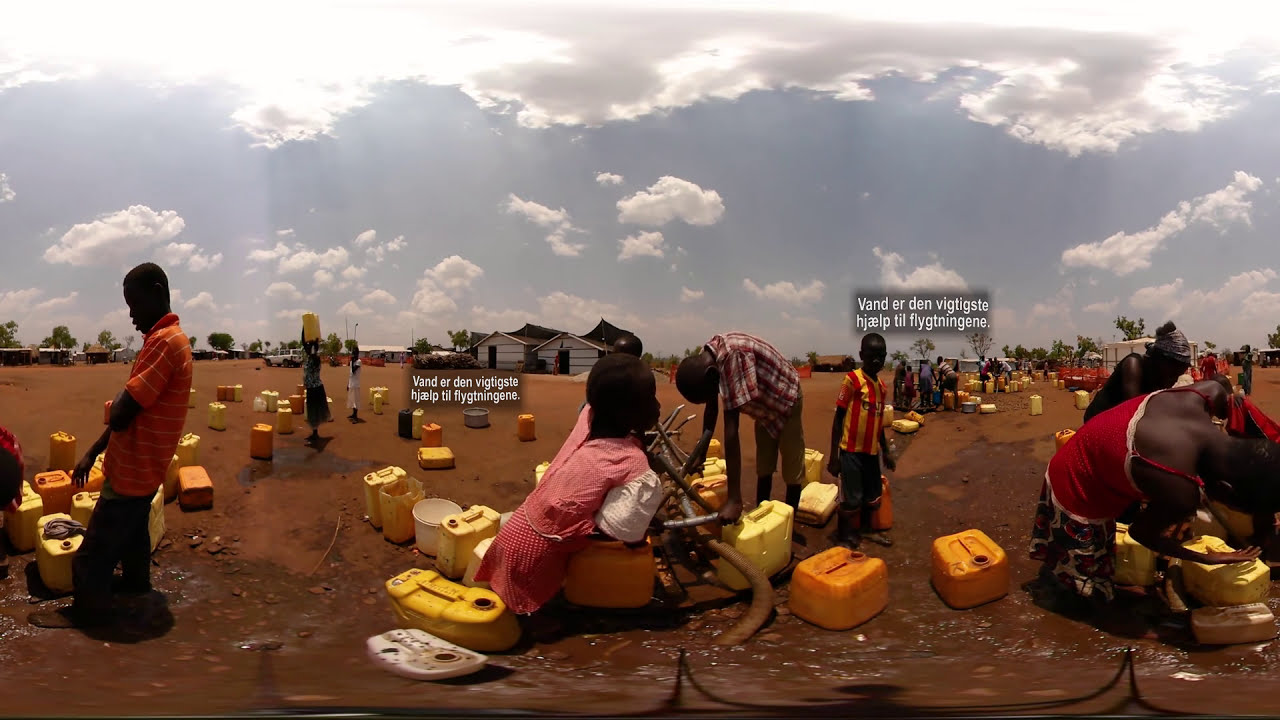In this photo, a group of dark-skinned individuals is engaged in various activities outdoors on a copper-colored dirt surface scattered with different colored pails and containers. Some people are sitting, others are standing or bending over, while several individuals are holding or carrying yellow and orange jugs, possibly for water. The sky above is blue with some clouds. In the background, there is a small shack-like building, alongside some other structures off to the left. Some of the people are dressed in traditional dresses, while others wear t-shirts. Foreign handwriting in white letters appears on some of the containers, though it is not readable. The scene appears to be set in a foreign country, likely outside in the middle of the day, giving the impression of people working or gathering in a communal effort.